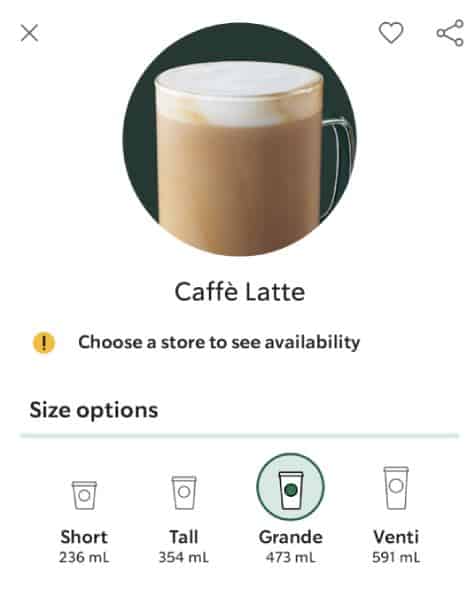The image displays a detailed product page for a café latte set against a solid white background. Central to the image, there is a round, color photo of a café latte in a clear glass cup with a silver handle on the right, featuring a mocha-colored drink topped with thick white foam. This cup is presented against a black background. In the upper left corner of the image, a small 'X' icon is visible, while the upper right corner includes a share icon and a heart icon. Beneath the café latte image, large bold text reads "Café Latte," and below that, in smaller text, it says "Choose a store to see availability." To the left of this smaller text is a small yellow circle with an exclamation point inside it. Further down, the image lists size options: Short, Tall, Grande, and Venti, with "Grande" highlighted and circled in green. Each size option is accompanied by an icon representing a cup of the corresponding size.